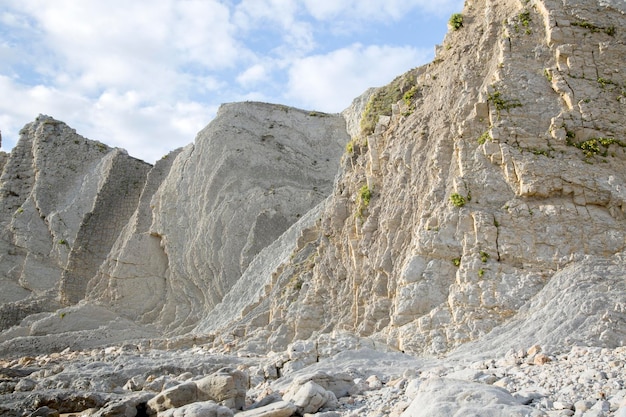This outdoor daytime photograph captures a rugged, rocky landscape dominated by a tall, jagged bluff that stretches horizontally across the image. The bluff, appearing approximately three to four stories high, showcases a mix of beige, light gray, and tan hues, with additional textured details like indentations and smooth surfaces. Sparse green moss and vegetation add hints of life, especially on the rightmost section of the bluff. The sky above is a brilliant blue, interspersed with large, fluffy white clouds that cover more sky than the blue, yet still suggest a clear, sunny day. The foreground is littered with a variety of rock debris, including beige and gray stones, indicating natural rockfall and contributing to the challenging, uneven terrain. This scene could evoke the idea of a potential hiking or climbing area, with its rough pathways and the natural beauty of the clear day highlighted by the bright, cloud-decked sky.